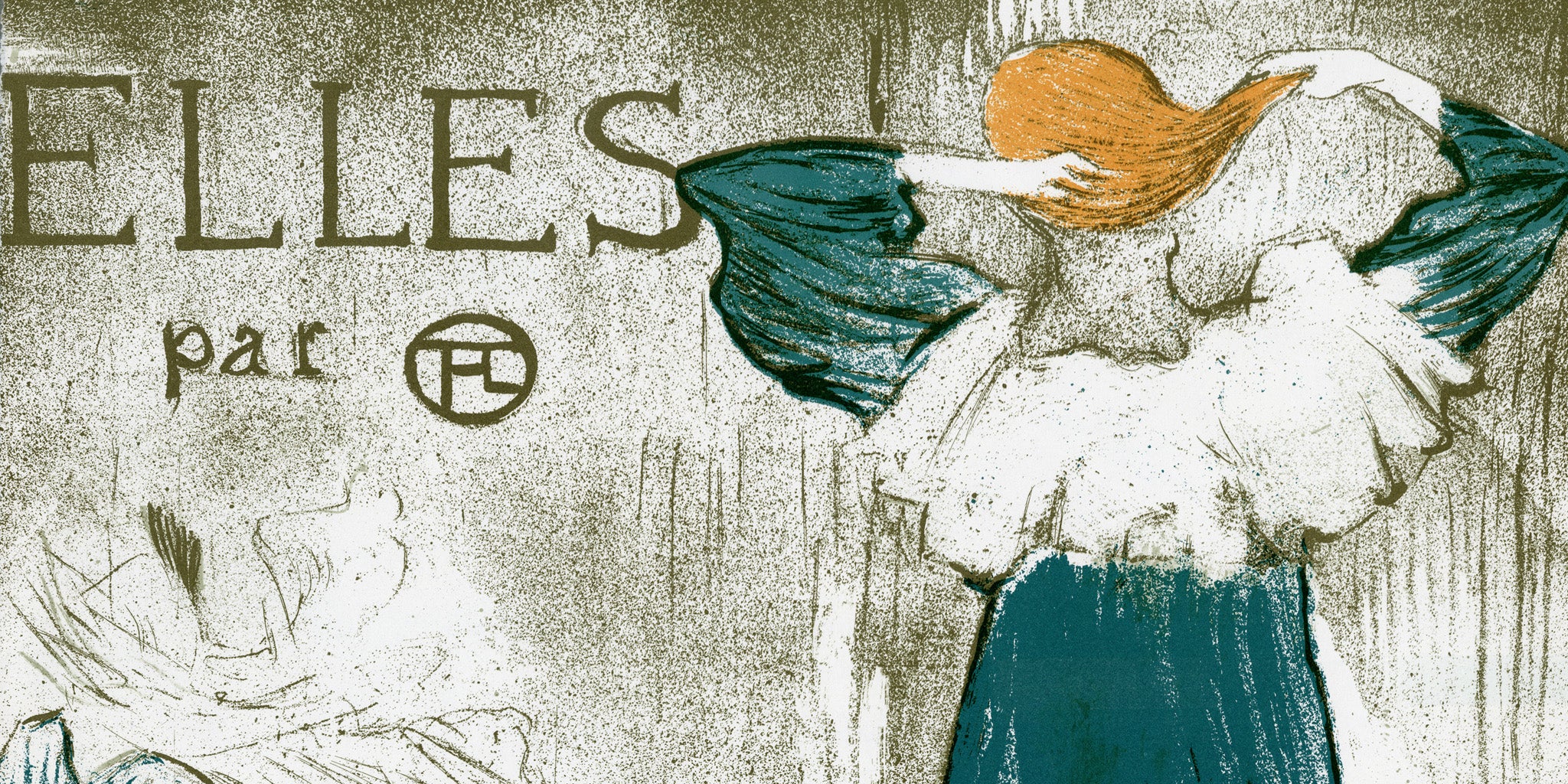This image is a detailed painting featuring a woman with striking red hair, possibly strawberry blonde, wearing a green dress with a distinctive white, bulbous upper part. She is depicted standing on the right-hand side of the image, seen from the back, with her left hand in her hair and her right hand pulling up the end of her hair, as if preparing to make a ponytail. The background of the painting is a textured white and brown, with areas of shading and green aging, suggesting an old, perhaps stone-like surface. At the top left of the painting, the text "L-E-L-L-E-S" is prominently displayed with "PAR" written smaller underneath it. Below this text is a circle containing the letters "FC". Additionally, there's an indistinct rough sketch at the bottom left, which could be interpreted as another figure or possibly even a representation of fire.